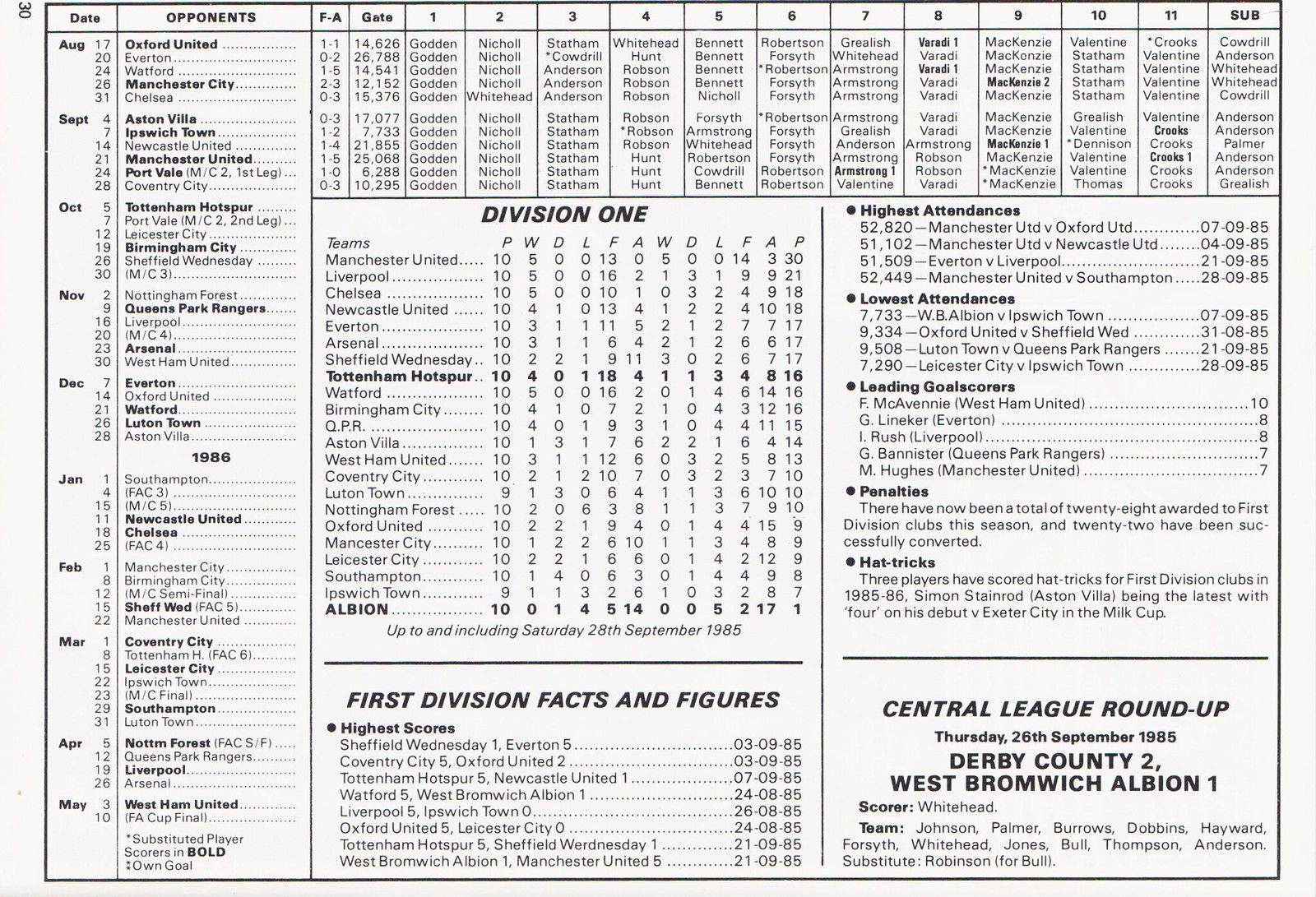The image is a highly detailed write-up for professional football (soccer) teams, covering the sports season from August to May. The left column lists dates, while the adjacent columns provide opponents' names, including prominent teams such as Oxford United, Manchester United, Tottenham, Birmingham City, Queen's Park Rangers, Arsenal, Everton, Watford, and Luton Town. This document is from 1986 and includes notable match information, player positions, and lineups. The top section specifies "FA Gate" with player names and numbers, indicating starting positions and substitutions: 1 (Golden, Nickel, Whitehead), 2 (Statham, Cowdrill, Anderson), 3 (Whitehead, Hunt, Robson), and so forth. The Substitutes section lists additional players like Cowdrill, Anderson, Palmer, and Grealish. The document also includes Division 1 team names and various statistics such as high attendance, low attendance, leading goal scorers, penalties, and hat tricks. The bottom right corner features a "Central League Roundup" for Thursday, 26 September 1985, detailing a match where Derby County defeated West Bromwich Albion 2-1, with Whitehead among the scorers and a lineup including Johnson, Palmer, Burroughs, and others.